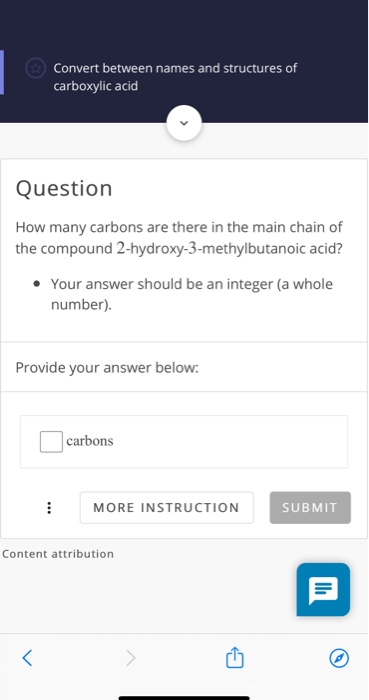This screenshot appears to be from a smartphone app designed to teach or test chemistry knowledge, specifically focused on organic compounds. 

At the very top, there's a blue text box with a title asking the user to "Convert between names and structures of carboxylic acids," accompanied by a down arrow button, likely for expanding additional information.

Below the title, a question reads: "How many carbons are there in the main chain of the compound 2-hydroxy-3-methylbutanoic acid?" 

A bulleted instruction specifies that the answer should be an integer (whole number): "Your answer should be an integer (a whole number). Please provide your answer below:"

The first option provided has a checkbox next to the word "Carbons," suggesting the user should type the number of carbons in the checkbox.

Below that option, there are two buttons: a white button labeled "More instruction" and a gray button labeled "Submit."

At the bottom of the screen, small text reads "Content attribution," and to the right of this text is a blue rectangular button with a speech bubble icon inside.

Finally, there are icons at the very bottom of the screen for navigation (back and forward), sharing, and opening the content in a browser.